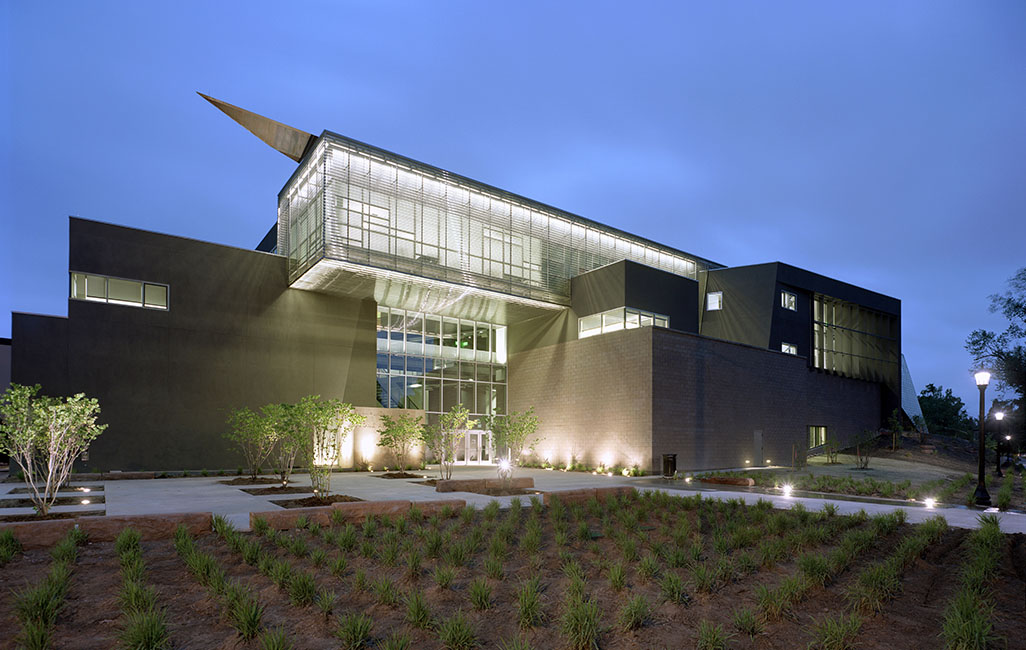This is an image of a large, contemporary office building, taken at dusk. The exterior is characterized by its modern, angular design, with no soft edges. The bottom floor is constructed from tan brick, while the upper floors feature extensive use of glass and possibly stucco. The ground floor includes a bank of four entry doors, leading into a two-story lobby that is fully glass-paned. The middle portion of the building is composed of cubic segments, creating a varied but cohesive architectural style. The left wing is mostly glass with a greenish hue and the right-hand side mirrors this with a similar color on the second floor. On the roof, there is a unique sculpture resembling a tipped spear or sword, matching the building's brown tones.

In the foreground, there is an immaculately landscaped courtyard with rows of neatly planted crops or shrubbery. Along the paths leading to the building are square sections housing illuminated trees, each space about five feet square. The surrounding walkways are lined with lantern-style street lamps and ground-level lights, adding to the building’s illumination. The photo captures the sky transitioning to dark blue, highlighting the building's bright interior and exterior lights, which cast a welcoming glow on the contemporary structure.